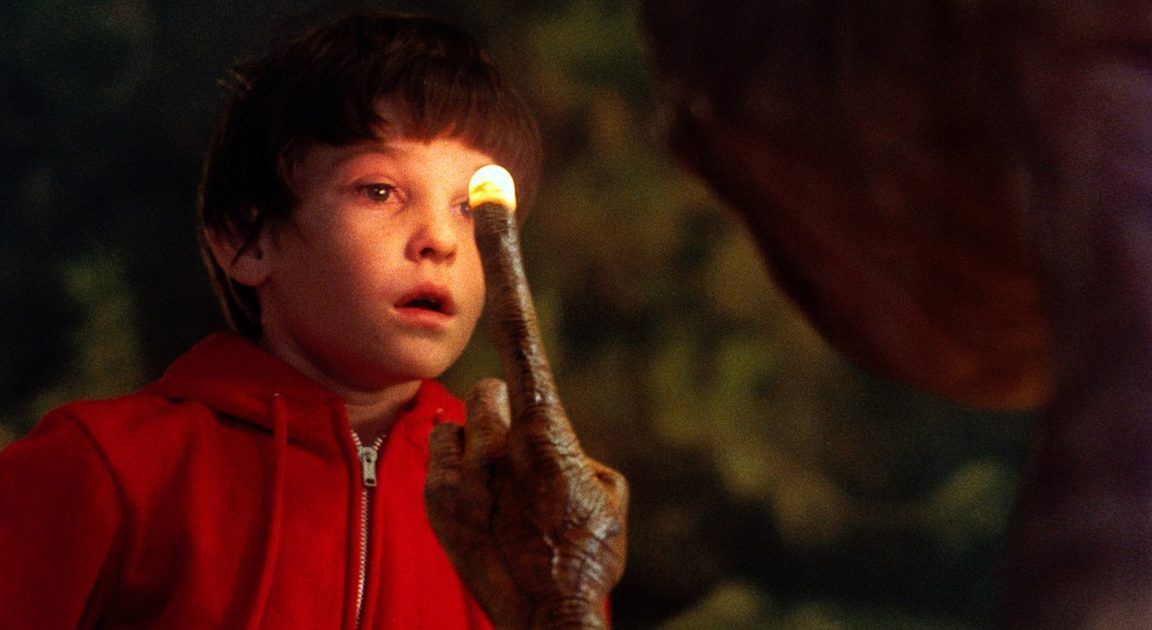The horizontally aligned rectangular image is a highly detailed and colorful scene from the movie E.T. It captures a pivotal moment where the young boy, wearing a zipped-up red hoodie, is staring in astonishment at E.T. His short brown hair is slightly combed over his forehead, and his mouth is open, reflecting his awe. The main focus of the picture is E.T.'s index finger, which is lit up at the tip and is positioned prominently in the center. The blurred, brownish outline of E.T.’s head is partially visible in the upper right corner, drawing attention to the boy's fascinated expression. The background, although blurry, displays shades of green and brown, hinting at bushes or trees. The natural light in the setting enhances the clarity of the image, emphasizing the boy’s expression and E.T.'s illuminated finger.